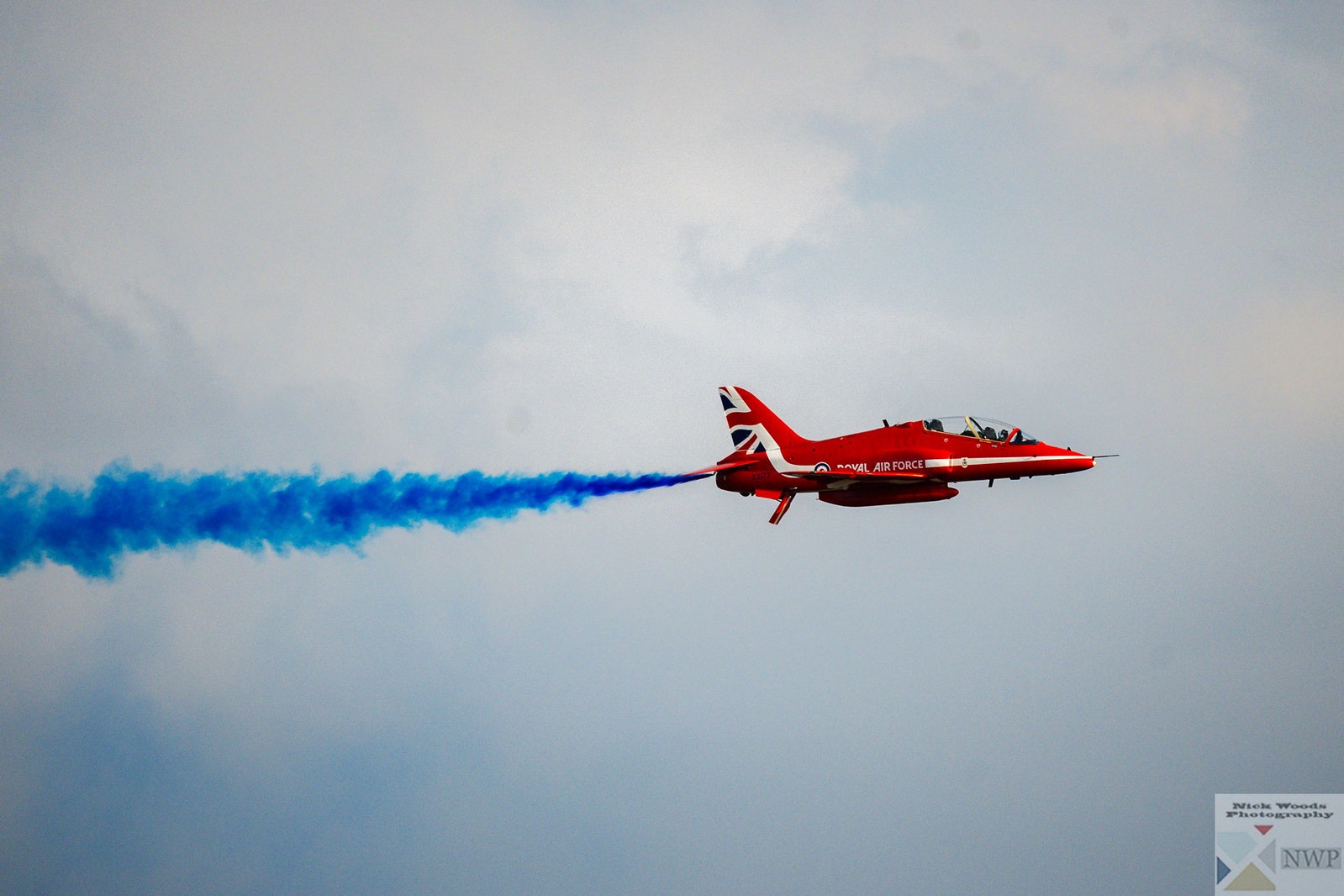This photograph, captured by Nick Woods Photography, features a red British fighter jet against a clear sky, creating a visually striking image. The jet's tail is adorned with the British flag, clearly identifying its origin. In the shot, the jet is releasing a distinct blue smoke or mist from its rear, possibly spelling out letters or forming patterns in the sky. The image effectively captures the close-up details of the aircraft and the vibrant blue smoke trailing behind it, showcasing a stunning aerial display.